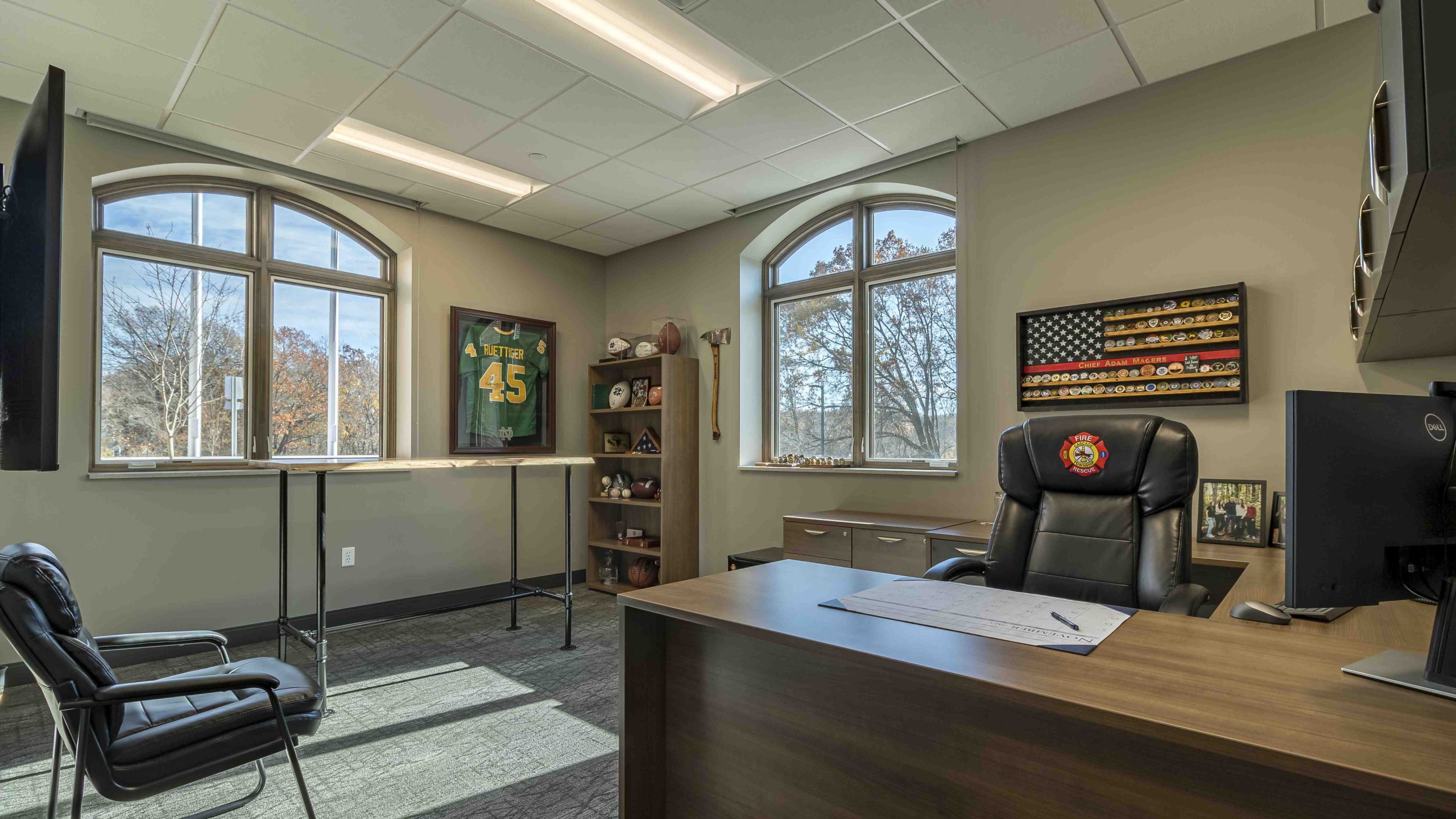The image depicts the detailed interior of an office, possibly belonging to a fire marshal or an executive with a strong affiliation to sports and patriotism. Dominating the room is an executive black leather chair embroidered with the insignia of a fire and rescue department. The backdrop reveals gray walls adorned with various items, including a prominently framed green and yellow football jersey featuring the number 45, which bears the University of North Dakota (UND) logo etched at the bottom. 

The left wall of the room hosts two large windows with curved tops, and an American flag rendered in artistic form hangs proudly. A collection of sports memorabilia, including footballs and baseballs encased in display boxes, is arranged on a shelf. Among these items, an axe is mounted on the wall, signifying a connection to either fire and rescue services or sports team trophies. 

Other furnishings include a sleek wooden desk, a computer set up with a monitor, mouse, and keyboard, and steel gray cabinets. The ceiling is outfitted with white tiles and long lamps for lighting. This meticulously arranged space, with its blend of professional and personal touches, reflects the importance and esteem of its occupant.